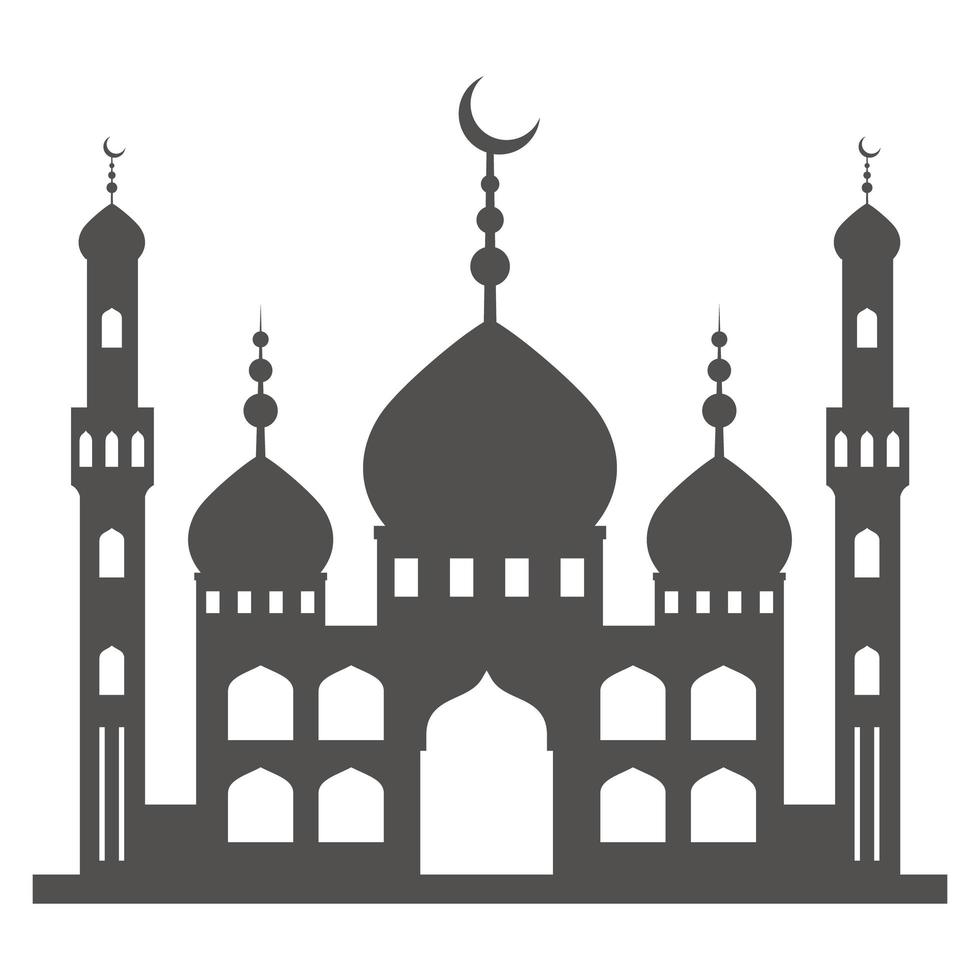The image depicts a simple, monochromatic graphic of a grand, Middle Eastern-style palace set against a white background. The palace is rendered in a dark gray or charcoal color and is presented as a flat, silhouette-like shape without intricate details. The central building features a large dome crowned with a tall spire ending in a crescent moon. Flanking the main dome are two slightly smaller domes that share a similar design but lack the crescent moon embellishment. The façade of the building is adorned with several rectangular windows that have pointed tops, giving it a distinctive architectural character. On either side of the central structure, there are tall, slender towers, each capped with narrow domes and smaller crescent moons. These towers also feature tall, pointed windows ascending their lengths. The overall impression is one of a majestic, yet simply illustrated, Middle Eastern palace or temple with iconic features like domes, spires, and crescent moons.